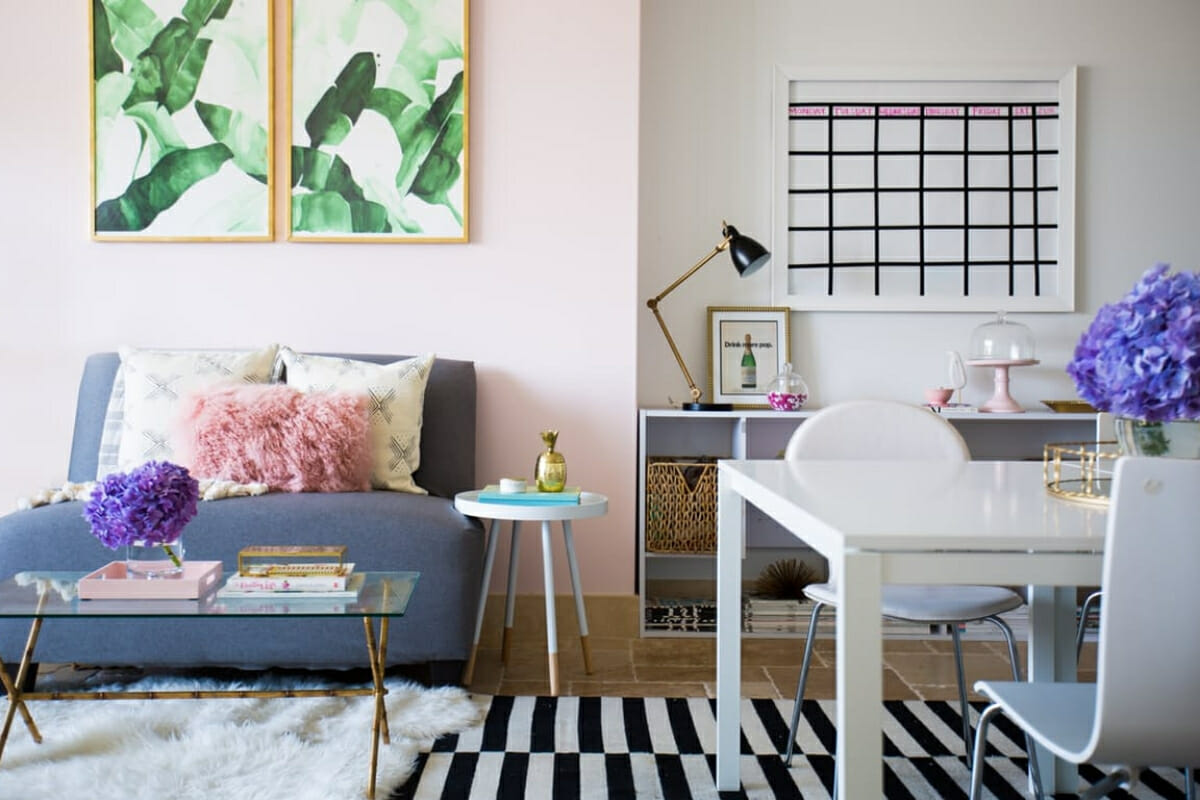This photograph captures a bright and meticulously arranged living area with walls in light pink and white hues. On the left side of the room, beneath two white-framed paintings featuring green leafy patterns, there is an armless blue-gray loveseat adorned with two patterned white pillows and a fluffy pink pillow. Adjacent to the loveseat, a small round white side table holds a few miscellaneous items. 

In front of the loveseat, a gold-legged glass coffee table hosts a stack of books and a jar of purple flowers. This coffee table sits atop a white shag rug, which itself is layered over a larger black and white striped area rug that partially covers the tiled floor. 

On the right side of the room, a dining area features a white table surrounded by white chairs, with a vase of purple flowers as its centerpiece. Behind the dining table, a whiteboard calendar hangs on the wall above a low white bookshelf adorned with a black lamp, photographs, decorative vases, and storage baskets on its lower shelves. The entire room exudes a clean and uncluttered ambiance.